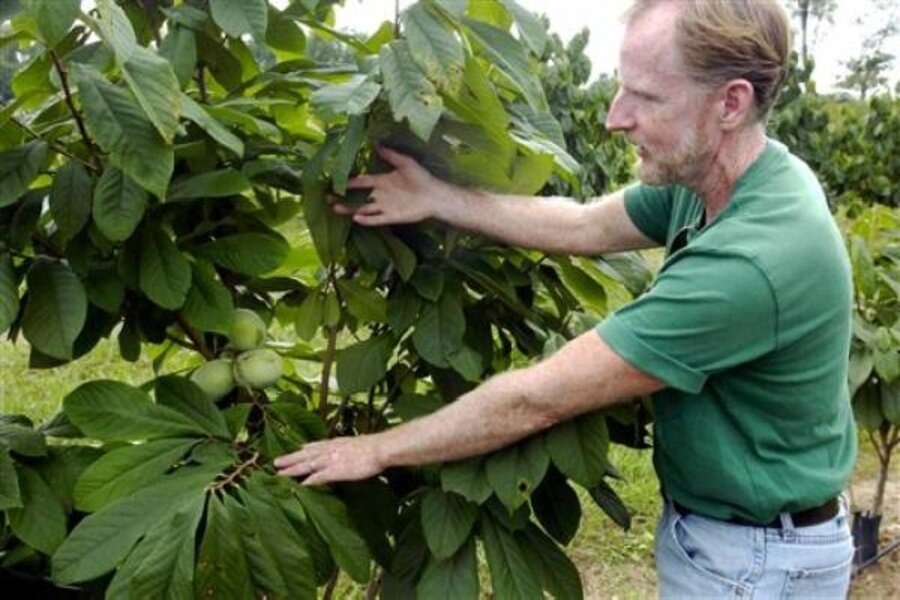In this photograph, a Caucasian man, likely in his late 50s to early 60s, is showcased standing outdoors amidst a scene of lush greenery. He sports short, red hair with a touch of gray, particularly in his beard and mustache, and has a prominent, pointy nose. He's dressed casually in a short-sleeved green shirt, light blue jeans secured with a brown belt, and he wears a wedding ring on his left hand, indicating he might be married.

The man is engaged with a fruit tree, pressing down some branches with his left hand and holding back others with his right, ensuring a clear view of the fruit for the photograph. The tree is abundant in green leaves and bears what appear to be green apples—three of which are visible in the center of the image. The background reveals more trees and patches of brown grass, under a white, overcast sky, adding a serene, pastoral ambiance to the scene. This setting suggests that the man may be on a farm or perhaps in a spacious backyard orchard.